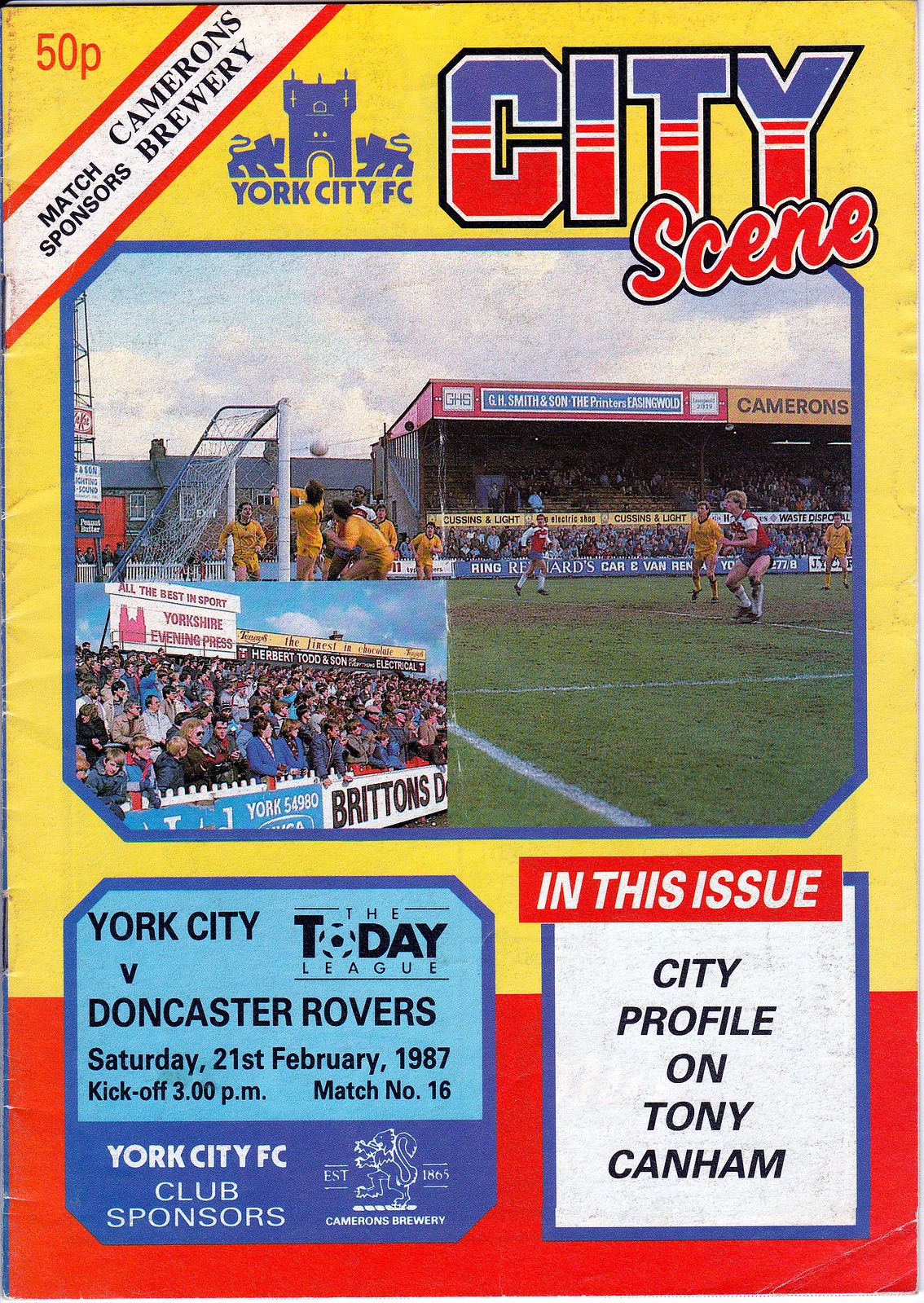The image is an old soccer program cover, predominantly featuring a bright yellow background on the top two-thirds and a red background on the bottom third. In the upper left corner, "50P" is printed in red. A diagonal white banner outlined in red, located just below, reads "Match Sponsors Cameron's Brewery" in black text. To the right of this banner, a blue emblem of a castle flanked by two lions prominently displays "York City FC" beneath it in blue text. Adjacent, in large, vibrant letters combining blue and red with outlines in black and white, is the title "City Scene," with "City" presented in block letters and "Scene" in red cursive.

Below the title, a photograph outlined in blue depicts a collage of soccer action: players in yellow and red/white uniforms on the field, and spectators in the stands. Beneath this image, to the left, a blue advertisement with black text reads "York City versus Doncaster Rovers at the Today League, Saturday 21st February 1987, kickoff 3 p.m., match number 16." Below, in dark blue with white print, it states "York City FC club sponsors." To the right of this section, a rearing lion beside the text "Established 1865" and "Cameron's Brewery" signifies the sponsor's history. The bottom right corner features a white square bordered in blue, containing the text "City Profile on Tony Canham" under a red banner stating "In this issue."